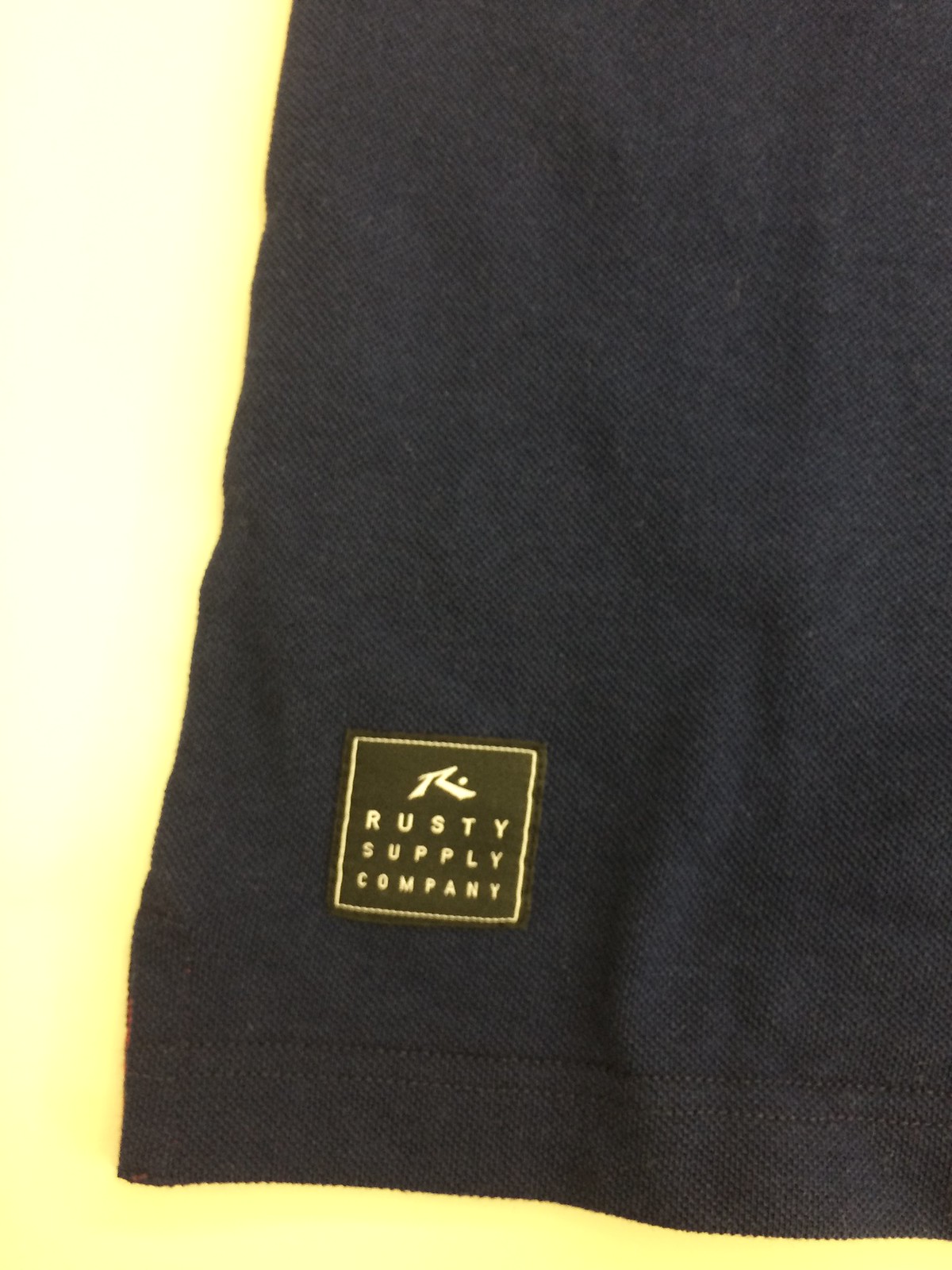The image showcases a detailed close-up of a piece of clothing or fabric. The background on the left-hand side and the bottom portion features a gradient of yellow, with the hue appearing much lighter towards the left and transitioning to a deeper, more saturated yellow at the bottom. Dominating the right-hand side of the image is a dark blue, nearly black piece of fabric. Near the bottom-left corner of this fabric, there is a small black square with neatly stitched white borders. Inside the square, there is a prominent white letter "R" along with the words "Rusty Supply Company" inscribed in white, neatly stacked beneath the large "R". The precise white stitching and the clear, bold font of the text contrast sharply against the dark fabric, making the branding distinctly visible.